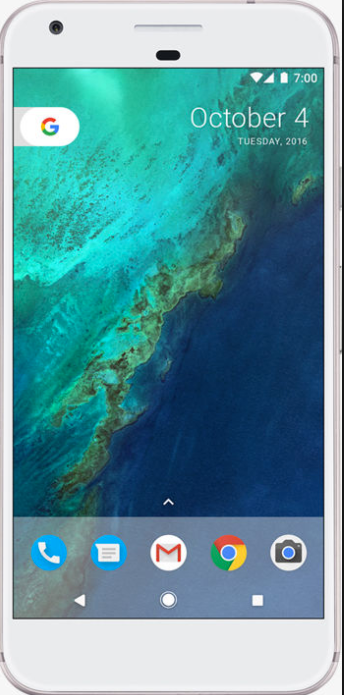This image depicts a screenshot of an older model white iPhone, characterized by distinct white bands on the top and bottom of the device. The screen displays a vibrant scene featuring a body of water with surrounding land, showcasing hues of blue and green. 

In the upper right corner of the screen, icons indicate full Wi-Fi and cell signals, alongside a battery icon reading 7:00 AM. On the upper left, a colorful banner with a capital "G" represents the Google logo.

Adjacent to it on the right, the date is clearly displayed: "TUESDAY, OCTOBER 4, 2016." A transparent banner spans the bottom of the screen, featuring an upward-pointing arrow above it. Within this banner, several icons are visible: a phone icon in a blue circle, a blue text bubble, an envelope symbol for email within a circled "M," the Chrome browser icon, and a circular camera icon. This intricate layout offers a snapshot from a specific moment in time, complete with app shortcuts and essential phone indicators.